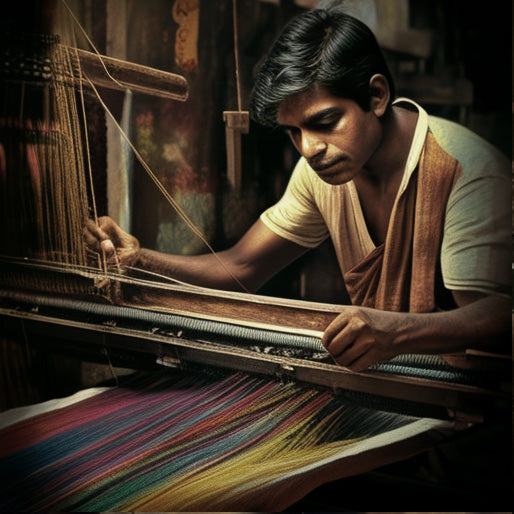In the AI-generated image, an Indian man works at a large loom, methodically weaving various colorful strands of yarn. The scene is illuminated by harsh overhead lighting, casting stark shadows that create dramatic contrasts and lend a visually intriguing quality to the image. The man, wearing an orange and beige shirt that blends oddly with his sash, appears detached from his meticulous task, possibly bored. His black hair, parted on the side, complements his brown skin. The vibrant yarns—ranging from pink, red, blue, orange, green, to yellow—are set against a backdrop of muted purples, teals, maroons, and burgundies, producing an almost rainbow-like ambiance. Despite the detailed rendering of threads in various shades, an AI-generated anomaly is apparent: the man's arm is not correctly connected, and his shirt’s structure is nonsensical. The setting, dimly lit with a focus on the loom, suggests a dark interior, adding to the aura of tedious handiwork in a shadowy, indeterminate environment.